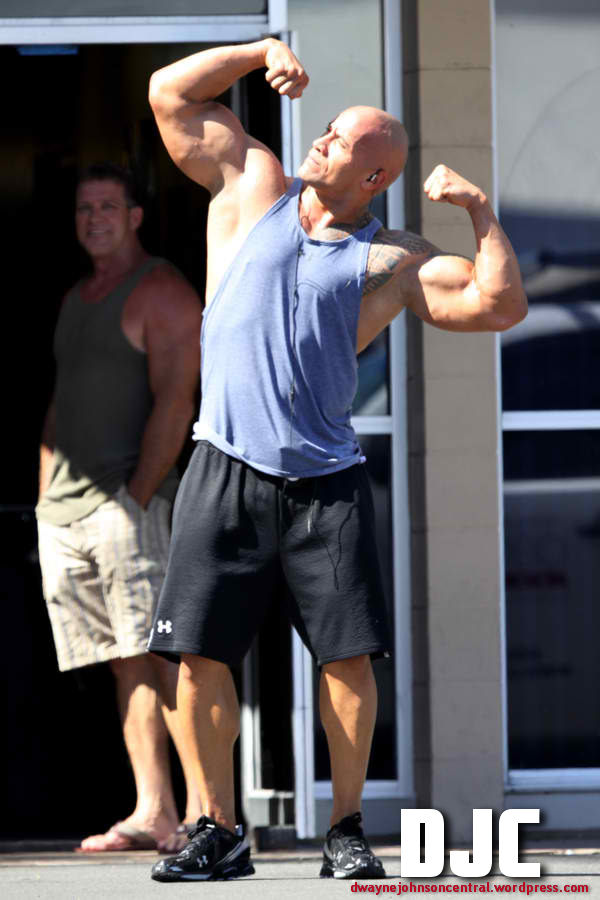In this photograph captured on a sunny day, a well-toned, bald man stands prominently in the center. He is mid-flex, showing off his biceps while looking towards the top left corner of the image. This bodybuilder is wearing a sleeveless blue tank top with deep-cut sides, black Under Armour basketball shorts, and black sneakers featuring white stripes on the sides. Black music earbuds are visible in his ears. His pose emphasizes a tribal tattoo on one of his shoulders. Behind the central figure and slightly to the left stands another man, sporting a sleeveless green t-shirt, gray shorts, and tan sandals, with both hands tucked into his pockets, and positioned in a doorway. Overlaying the photograph, the letters "DJC" are printed in bold white text, with "drainjohnsoncentral.wordpress.com" written below in smaller red font. The bright sunlight illuminates the scene, suggesting it might be outside a gym.